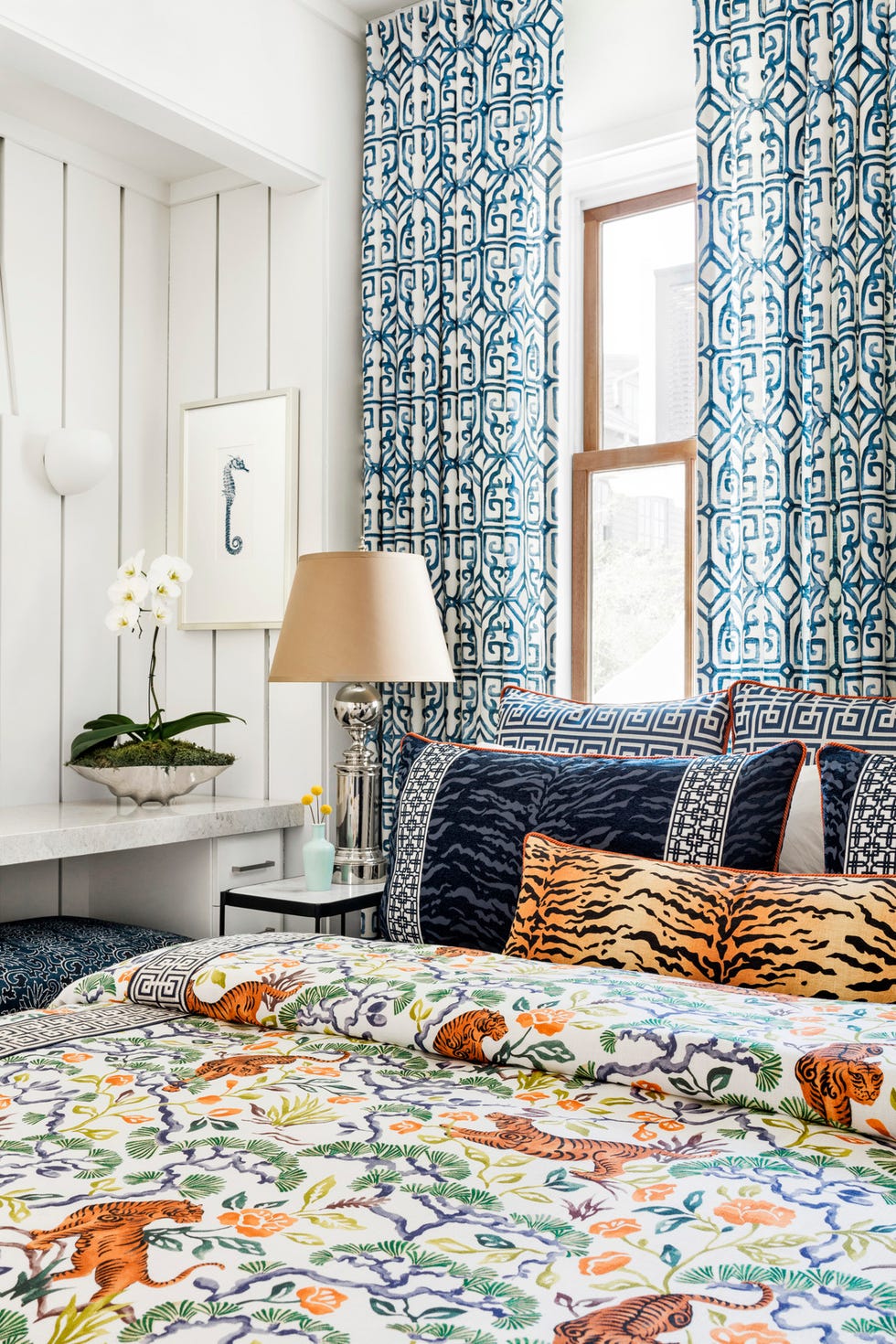This is a beautifully lit bedroom, bathed in natural light from a large window framed in tan, located behind the bed. The room has white shiplap walls that enhance its airy atmosphere. The bed is adorned with a vibrant comforter that depicts a jungle scene, featuring tigers and various flora against a white background. This comforter is complemented by an array of pillows, including a long oblong tiger print pillow set in front, flanked by blue sham pillows, and white pillows at the back. 

The intricate window curtains showcase a teal and cream design that adds to the room's coastal ambiance. To one side of the bed, there is a small night table holding a lamp with a beige lampshade atop a silver base, accompanied by a smaller vase with yellow flowers. A little desk nook on the opposite side offers functionality, adorned with a framed seahorse image and a bowl of orchids. Little stools tucked under the counter provide additional seating options. Overall, the room is a harmonious blend of vibrant patterns and serene coastal elements, resulting in a light, bright, and colorful space that feels both dynamic and serene.